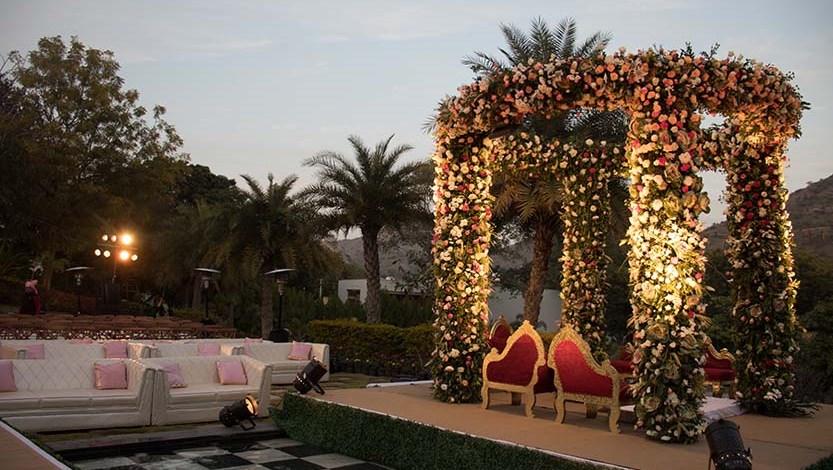This photograph captures an enchanting outdoor event venue during the evening, believed to be in a warm climate as indicated by the presence of palm trees. The scene is set in an open-air space, possibly a backyard, condo, or resort area. In the bottom left corner, a black and white checkerboard pattern tiles the ground, indicating part of a dance floor or seating area. Adjacent to this is a series of white couches or loveseats, adorned with pink throw pillows, arranged in multiple rows leading towards a grand stage.

The stage, positioned slightly elevated, features a green front that resembles grass, with numerous spotlights illuminating its structure from various angles. Dominating the stage is a magnificent floral gazebo-like structure. This flowered gazebo is supported by four green pillars completely enveloped in white and pink flowers and grasses. The top of the gazebo, forming a circular canopy, is also richly decorated with these flowers, creating an enchanting and romantic atmosphere reminiscent of a wedding setting. Within the gazebo, several red and gold chairs are arranged, adding a touch of opulence.

Behind the stage, the serene setting continues with a backdrop of trees and a clear blue sky. On the left, a small building and some lights are partially visible, and in the distance, a large palm tree stands prominently, surrounded by more vegetation and possibly additional structures or a hedge. To the right of this, a trail of smaller palm trees and another building in the far distance contribute to the overall picturesque setting. The ambiance is further enhanced by the warm, inviting glow cast by the spotlights, creating a magical and serene evening atmosphere.